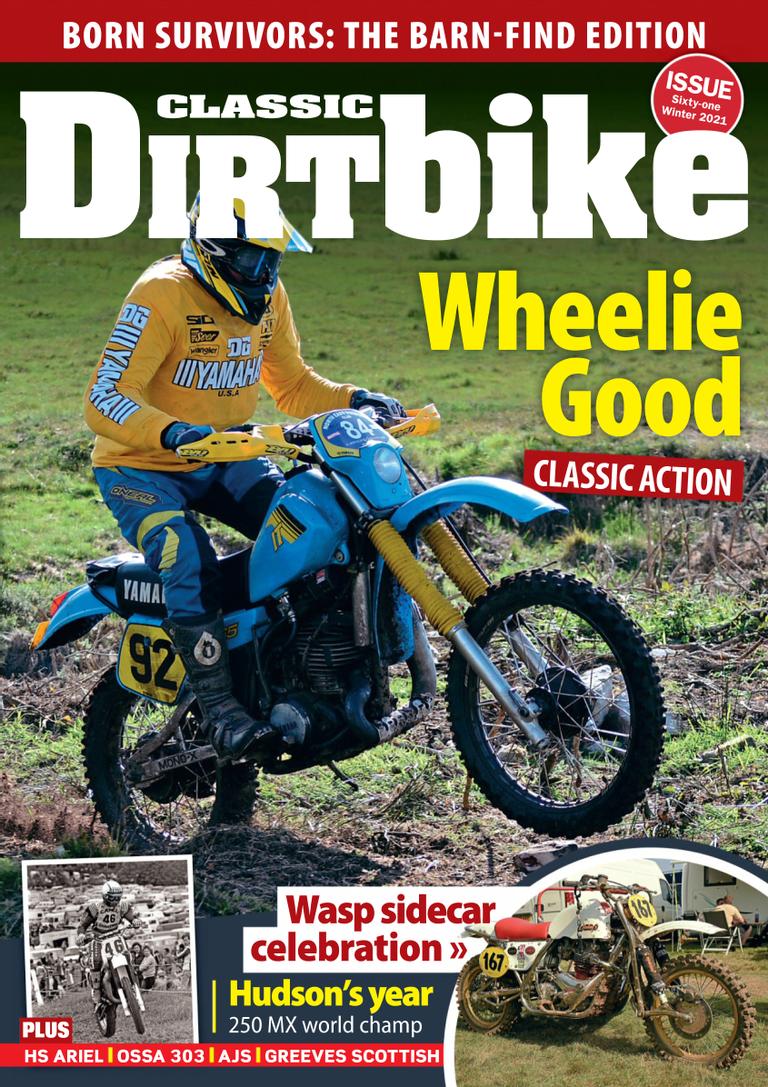The cover image of the magazine "Classic Dirt Bike" features a striking scene of a man performing a wheelie on a light blue and yellow Yamaha dirt bike marked with the number 92. The rider is clad in a coordinating outfit, including a yellow long-sleeve t-shirt with white lettering, likely saying Yamaha, blue and yellow pants, and a matching helmet. The top banner of the magazine, in a bold red, announces "Born Survivors, the Barn Find Edition." Below this, the main title "Classic Dirt Bike" is prominently displayed in white, followed by the subtitle "Wheelie Good, Classic Edition."

The lower portion of the cover features additional intriguing elements. On the lower left, there’s a black-and-white photo of another dirt bike rider, numbered 46, who is donned in a protective, armor-like outfit and a white helmet. On the lower right, a vintage, well-worn dirt bike with a red seat and the number 167 is showcased, adding to the nostalgic charm of the magazine. Captions such as "Wasp Sidecar Celebration" and a note on "Hudson Year 250 MX World Champ" hint at the rich, diverse content within the magazine.